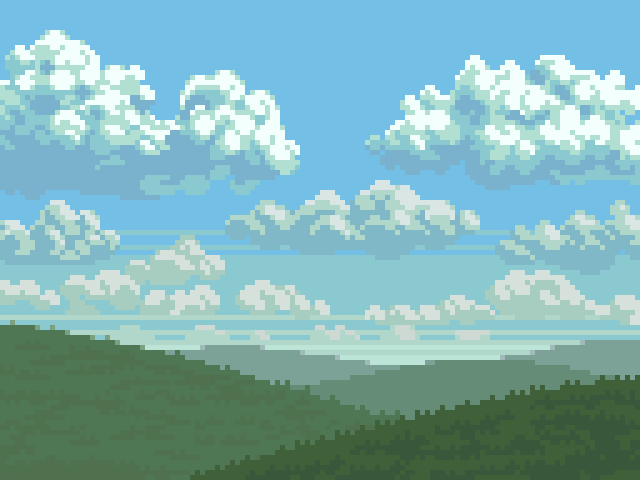The image is a highly pixelated, rectangular outdoor scene that resembles an early computer illustration, likely created with a limited color palette for stylistic effect. The foreground features two overlapping hills, with the bottom right hill being the darkest green and the bottom left hill a lighter green. There are three additional hills in the background that are progressively grayer. The sky, taking up the upper portion of the image, is a gradient from light to medium blue, populated by a variety of pronounced clouds. There are about eight to nine large clouds, with a mix of white, dark blue, yellow, and perhaps green hues. The pixelation is pronounced across the entire image, giving a clear view of individual squares used to compose the overall scene. The image lacks any human figures or the sun, emphasizing the abstract nature of the landscape.